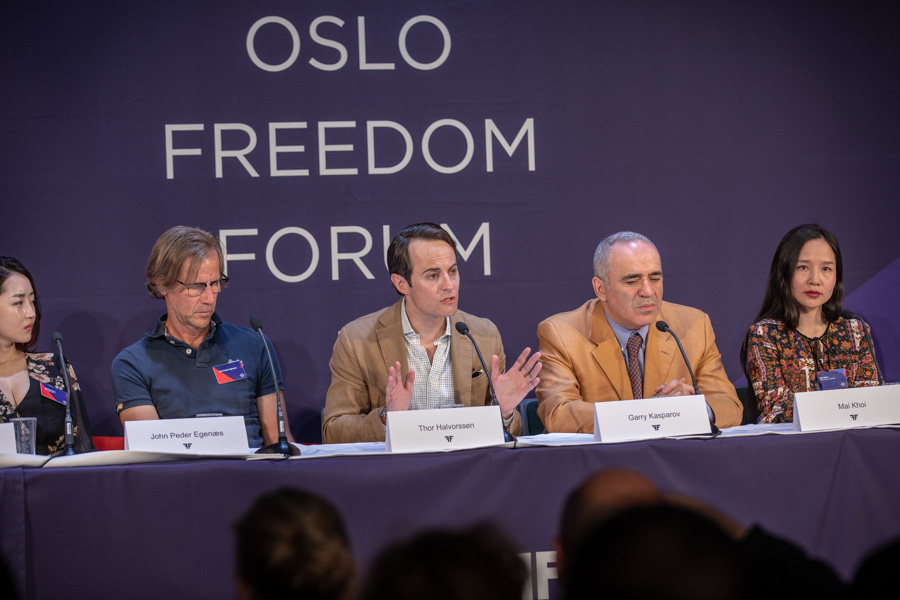The photograph depicts a panel of five individuals seated behind a table at the Oslo Freedom Forum, as indicated by white capital letters in the background. On the far left is an Asian woman dressed in a black dress. Beside her sits a man with long hair wearing a dark blue polo shirt with a red triangular logo. At the center of the group, a man dressed in a brown blazer over a blue shirt appears to be speaking, his mouth slightly open and hands raised, while the others attentively listen. To his right is a man in a dark orange t-shirt layered under a blue blazer. On the far right is another Asian woman in a black dress adorned with red triangular designs. Each panelist has a name card and microphone in front of them, though the names are too small to discern. In the foreground, an audience sits, engaged with the ongoing discussion.